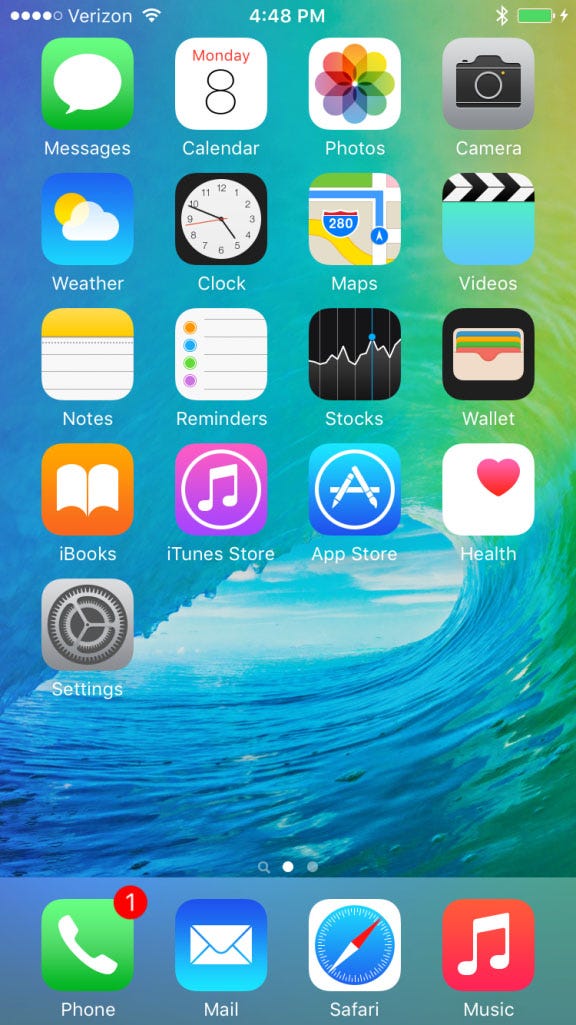This image captures a detailed view of a smartphone home screen interface. At the top of the screen, there are four white signal dots out of a possible five, indicating network strength under the “Verizon” title. The time displayed is 4:40 PM, with a fully charged battery icon beside it.

Below the top bar, various application icons are arranged in rows. The first row includes the following icons and their descriptions:
- **Messages**: Represented by a speech bubble icon.
- **Weather**: Depicted with a cloud and sun icon.
- **Notes**: Symbolized by a white paper with a yellow header.
- **iBooks**: Shown with a book icon.
- **Settings**: Displayed with a gear icon.

The second row of icons includes:
- **Calendar**: Highlighted on Monday the 8th.
- **Clock**: Indicating the time as 5:50 PM.
- **Reminders**: Featuring an icon with orange, blue, green, and purple ovals and lines for input.
- **iTunes Store**: Depicted with a musical note in a white circle.
- **Photos**: Shown with a multi-colored flower icon.
  
The third row contains:
- **Maps**: Illustrated with a map and the number 280.
- **Stocks**: Displayed with fluctuating line graphs.
- **App Store**: Represented by an "A" in a white circle.
- **Camera**: Shown with a camera icon.
- **Videos**: Depicted with a clapboard icon.
- **Wallet**: Illustrated with a wallet icon.
- **Health**: Represented by a heart icon.

This organized layout of icons provides a clear overview of the smartphone’s main applications and their respective visual representations.